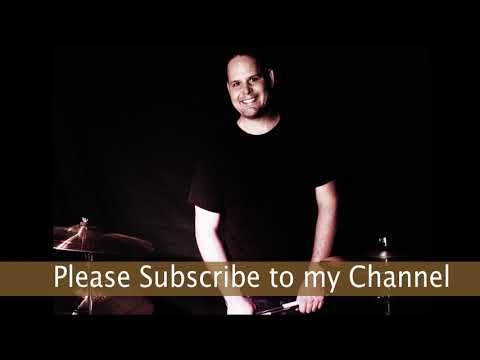The image appears to be a slightly blurry screenshot or thumbnail from a video, likely sourced from a platform like YouTube or Twitch. The central figure in the image is a smiling man with white skin, dark hair, and dressed in a black short-sleeve T-shirt. He appears to be a drummer, as he is holding drumsticks and there are symbols indicative of a drum set visible around him. The background behind the man is predominantly dark, featuring shades of black and dark brown, which might be fabric or other backdrop materials. At the bottom of the image, a light brown horizontal banner spans across, displaying the text "Please subscribe to my channel" in white letters. The surroundings of the image are mostly black, enhancing the emphasis on the central figure and the subscription request.